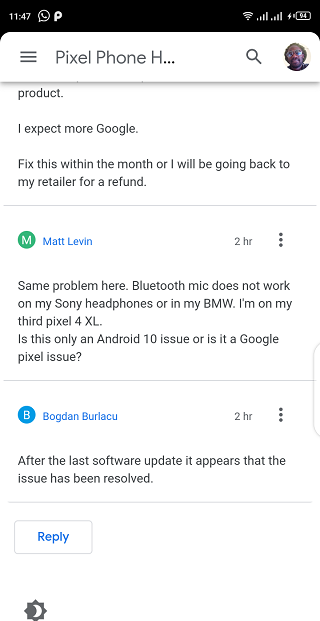A detailed screen grab of a Google Pixel phone capturing a user's text or social media conversation. The image shows the phone interface with a horizontal black bar at the top displaying the time "11:47" in white on the left side. A white speech bubble icon containing a receiver and a dense white "P" are positioned next to it. To the right, there is a Wi-Fi signal indicator, two sets of four signal bars each, and a battery icon showing a 94% charge level.

Below the black bar, the app interface includes three horizontal lines on the upper left for a dropdown menu, the text "Pixel phone H..." in gray at the center, a magnifying glass icon for search, and on the far right, the user icon of a middle-aged man with longish curly hair, glasses, and a thick mustache.

The first section of the conversation reads: "Product. I expect more Google. Fix this within a month or I will be going back to my retailer for a refund."

The next message, identified by a green icon with a white "M" and labeled "Matt Levin" in blue, states: "Same problem here. Bluetooth mic does not work on my Sony headphones or in my BMW. I'm on my third Pixel 4 XL. Is this only an Android 10 issue or is it a Google Pixel issue?" This was posted two hours ago.

Following that, another message from "Bogdan Berlikow" in blue, also posted two hours ago, says: "After the last software update, it appears that the issue has been resolved."

A gray horizontal line separates the messages, with a gray outlined button labeled "Reply" and a brightness indicator located on the left side of the screen.